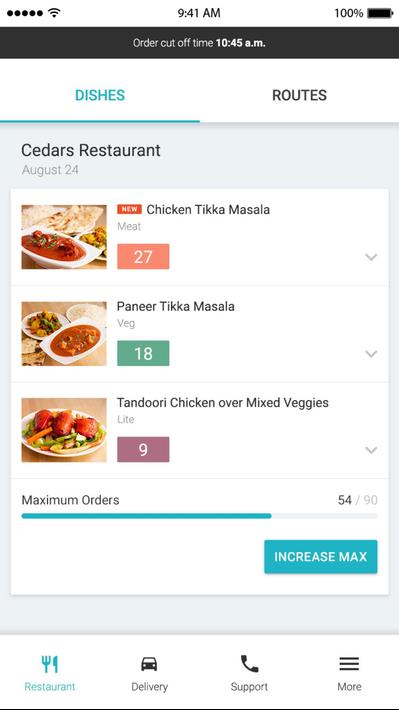This screenshot, taken from a cell phone, prominently features a predominantly white background. At the top, you can see standard phone status indicators including the time (9:41 AM), a 100% battery icon, five horizontal dots indicating service strength, and an internet connectivity status symbol. Below this, a black banner displays the text "Order cutoff time, 10:45 AM," followed by a white banner highlighting navigation tabs labeled "Dishes" (highlighted in blue) and "Routes."

In the body of the image, which references Cedars Restaurant on August 24th, there are three horizontally-aligned sections, each with a white background and black text, detailed as follows:

1. **Chicken Tikka Masala (Meat)**:
   - Displayed with an image of the dish on the left.
   - The text "27" bordered in orange.

2. **Paneer Tikka Masala (Veg)**:
   - Accompanied by a dish image on the left.
   - The background is turquoise, with "18" displayed.

3. **Tandoori Chicken over Mixed Vegetables**:
   - Also includes a dish image on the left.
   - The background is purple, with "9" shown.

A note at the bottom of these sections reads "Maximum order is 54/90," with a blue button below saying "Increase max." At the bottom navigation bar, you can see options labeled "Restaurants," "Delivery," "Support," and "More," providing additional functionalities. The overall interface clearly outlines menu offerings and ordering details for efficient user interaction.